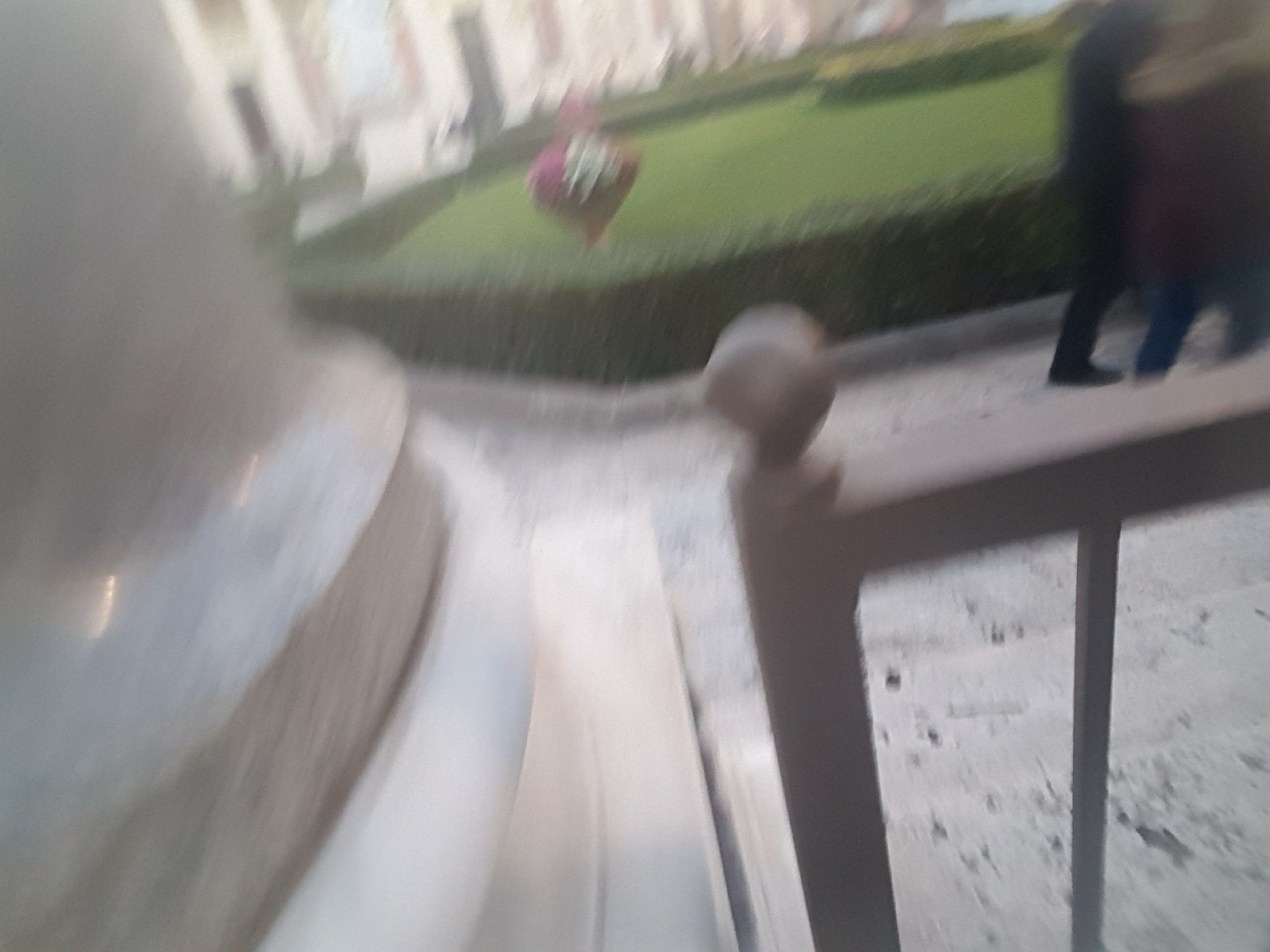This outdoor image, though slightly blurred, captures a picturesque scene. In the foreground, there's a short stone fence adorned with a vibrant bouquet of pink and white flowers. Behind the fence, a gently raised grassy area adds a touch of natural greenery. To the right, a light-colored concrete building stands tall, featuring a prominent concrete post. Adjacent to the building is a metal fence that lines a concrete walkway. Within the image, the faint outline of a man dressed in a black suit can be observed, accompanied by what appears to be another person in motion, their form blurred to the point of near invisibility. The overall composition presents a serene yet dynamic moment in a seemingly tranquil setting.